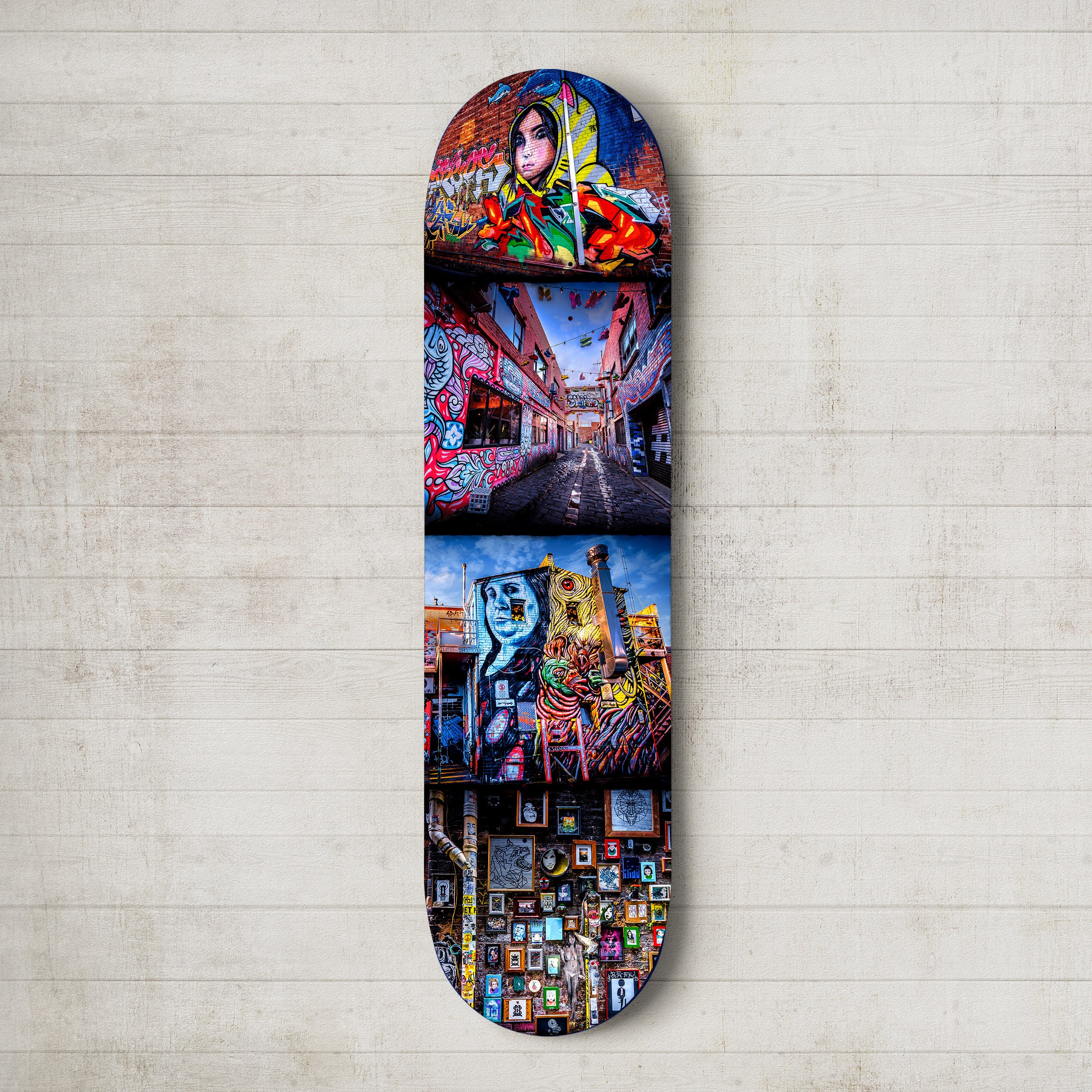The square photograph, measuring six inches by six inches, features a light gray wooden paneling background with horizontal slats about a quarter of an inch wide each. Centered within the image is a long, oval-shaped object, approximately five inches high and one inch wide, which could be a skateboard or surfboard-like item. This object displays vibrant, graffiti-like paintings divided into four distinct sections. 

At the top, there is a depiction of a young girl with black hair, wearing a yellow and gray striped hoodie with cat ears, facing to the left. The second section presents a street view, showcasing red-painted buildings adorned with blue fishes. The third section features tall buildings covered in multiple graffiti artworks, including a large blue face of an overweight person with black hair and a prominent red eye. The bottom section illustrates a wall filled with numerous small framed pictures.

The detailed artwork on the long oval object, whether hung or placed on the floor, highlights an eclectic mix of urban and whimsical elements, resonating with the dynamic essence of street art.